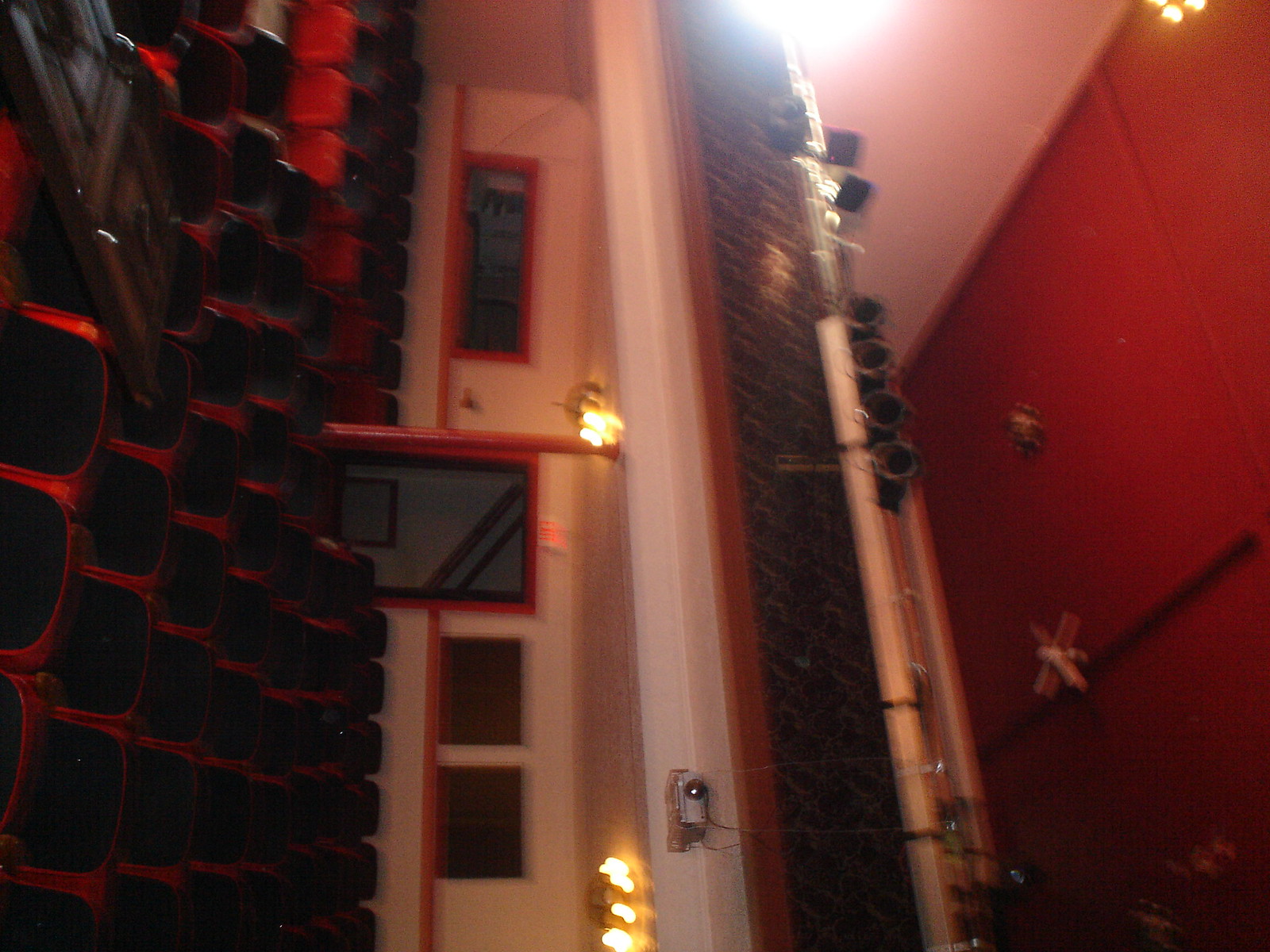This is a sideways photograph of an auditorium or movie theater, with the photo needing to be rotated to the left for proper orientation. The image captures the back seven or eight rows of black seats with red trim, arranged parallel to an aisle that runs down the center. This aisle appears to the left in the current sideways view. The white walls of the venue contrast with the reddish ceiling, which features a white ceiling fan and beams with attached black spotlights.

In the mid-background, long and short rectangular windows punctuate the wall. A balcony, with a black and brown railing and centrally mounted lights, is visible above the seating area. Below this balcony, a projector is affixed, aimed towards the seating. Additional lighting and a doorway with an exit sign are also visible beneath the balcony. The overall blurred quality of the photograph slightly obscures these details but provides a clear enough view to identify the key features of the theater.